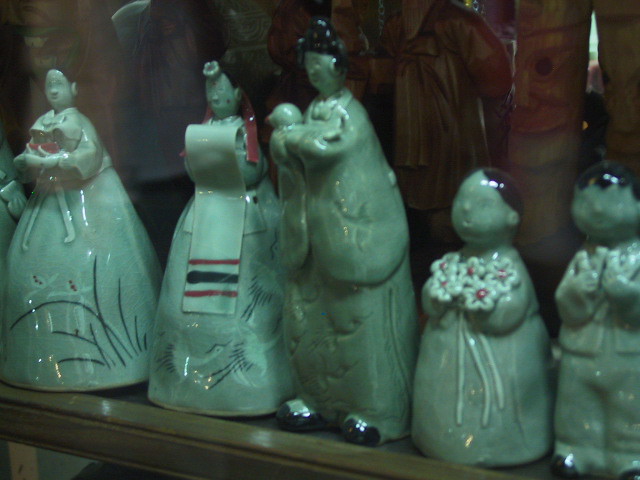The image portrays a collection of five glossy, ceramic figurines with a distinctly Asian influence, likely representing a family and crafted in a jade green hue. They are set against a dark, indistinct background and appear to be displayed on a shelf, suggesting a curated mantle or china cabinet arrangement. The figurines include three larger adults and two smaller children, each with intricate etchings or carvings on their surfaces. 

The adult figures, likely female, wear kimonos adorned with designs such as cranes, plants, and intricate patterns. One figure resembles a woman holding a small animal or baby, identified by her black shoes, while another appears to hold a scroll or possibly fruit. The third adult figure features etched grass and additional detailing. 

On the right side of the arrangement, the children are dressed similarly with one, a girl, clutching a bouquet of flowers, and the other, a boy, in a suit jacket and pants whose held item is less discernible. All the figurines have shimmering, defined facial features indicative of their porcelain craftsmanship, contributing to their overall ornate and collectible aesthetic.